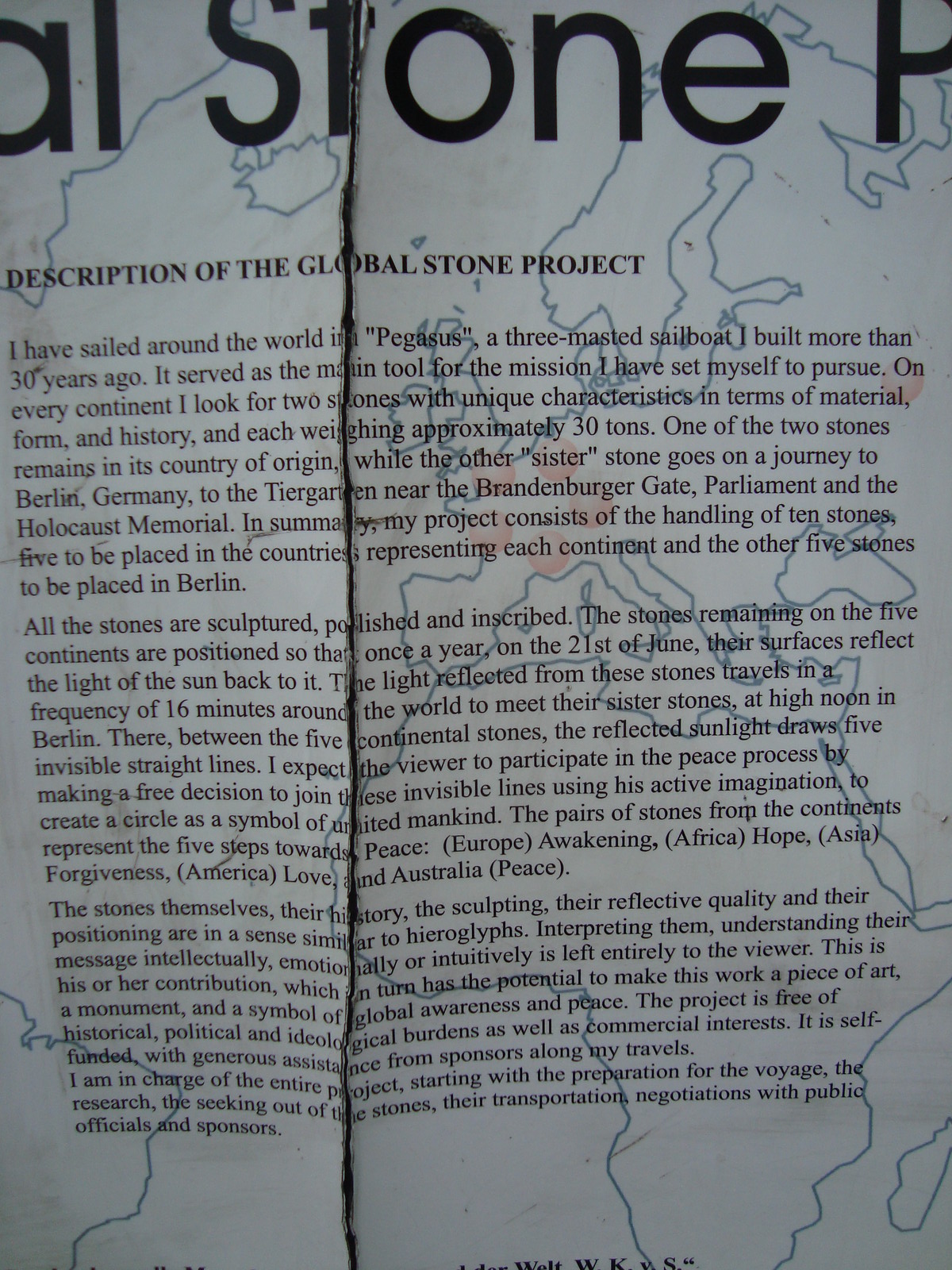The image features a torn and reassembled page, torn vertically down the middle, from a book or a booklet. The page details the title "Global Stone Project," written in bold black letters at the top, though partially obscured. Below the title are three paragraphs elaborating on the project. The page's background is light gray and showcases a blue outline map of the world, highlighting Europe, Africa, and other continents. Notable red circles mark locations in France and Russia.

The text explains that the author has sailed around the world in Pegasus, a three-masted sailboat built over 30 years ago, serving as a principal tool for the mission. On each continent, the author identifies two unique stones, each weighing approximately 30 tons. One stone remains in its country of origin while the other is transported to Berlin, Germany, placed near the Brandenburg Gate, Parliament, and the Holocaust Memorial.

Overall, the project involves ten stones, with five remaining on their respective continents and the other five installed in Berlin. These stones, sculpted, polished, and inscribed, reflect sunlight in such a way that on June 21st each year, the light travels for 16 minutes to reach Berlin, connecting the stones with invisible lines. This light arrangement aims to form a symbolic circle of united mankind, encouraging viewers to engage with the project and contribute to the peace process imaginatively.

The stones from each continent symbolize different steps towards peace: Africa represents hope, Asia forgiveness, America love, and Australia peace. The stones' reflective qualities and positioning suggest hieroglyph-like messages, left open to individual interpretation. The project avoids historical, political, and ideological biases, relying on self-funding and the support of generous sponsors. The author oversees every aspect, from the voyage preparation to the stones' placement and negotiations with public officials and sponsors.